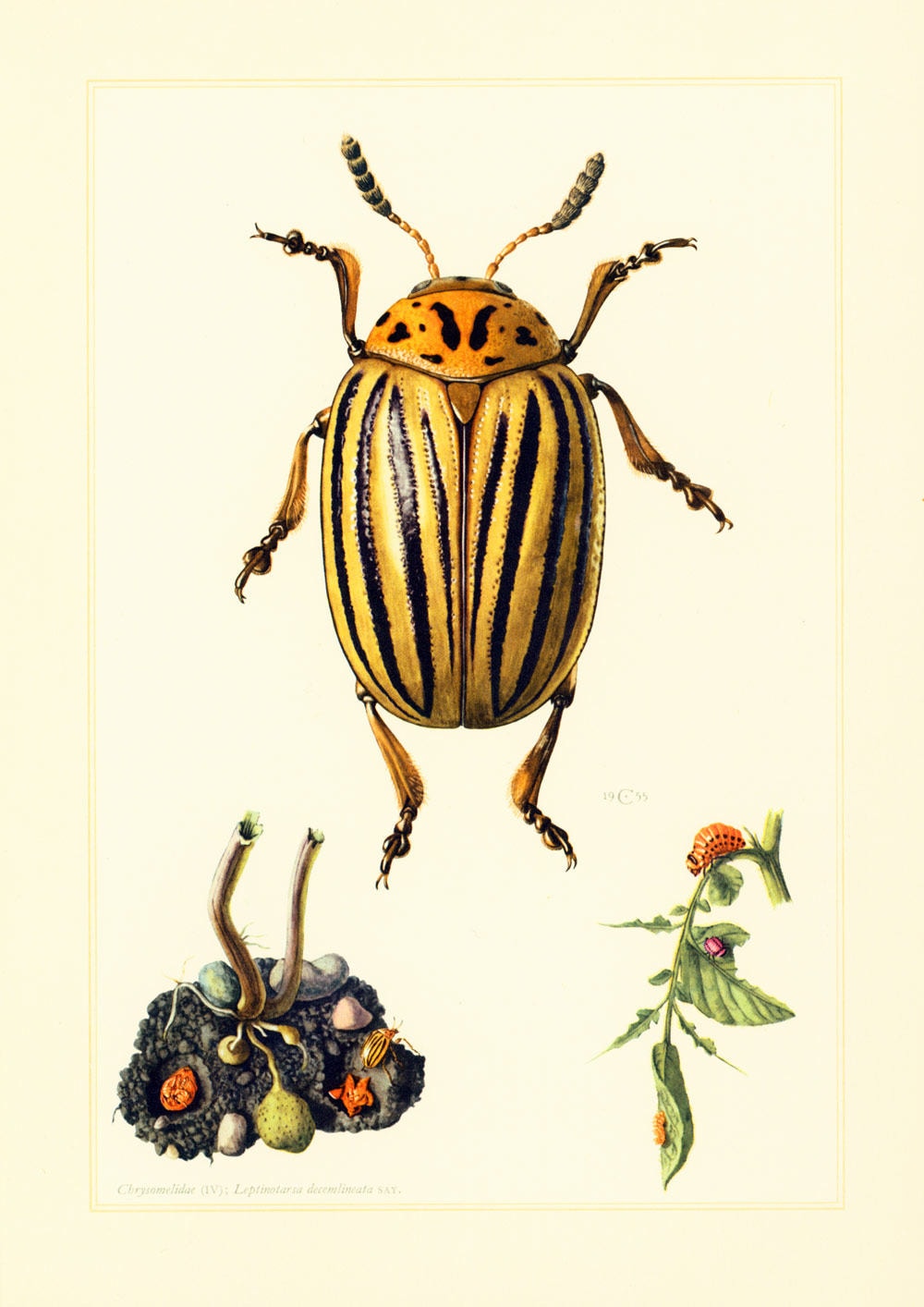The image prominently features a large beetle with a beige body and distinct yellow wings that have vertical black stripes. The beetle, positioned centrally and taking up most of the space, displays brown markings on its head and six legs. The background is a light pinkish-beige color, and there is a golden yellow square encircling the objects but not defining the outer frame of the image. 

Below the beetle, a pile of soil can be seen, appearing to have tentacle-like protrusions and colorful rocks scattered within it. There might be smaller beetles or other small organisms in the dirt, although they’re not clearly identifiable. To the lower right, a curving green plant features a red caterpillar-like creature climbing a vine, hinting at different life stages of insects present in the image.

Additionally, to the left of the beetle, there is a rock-like structure with various fungus growths, marked by orange and green shapes. The combination of these elements forms a rich and detailed depiction of a small ecosystem surrounding the central figure of the beetle.